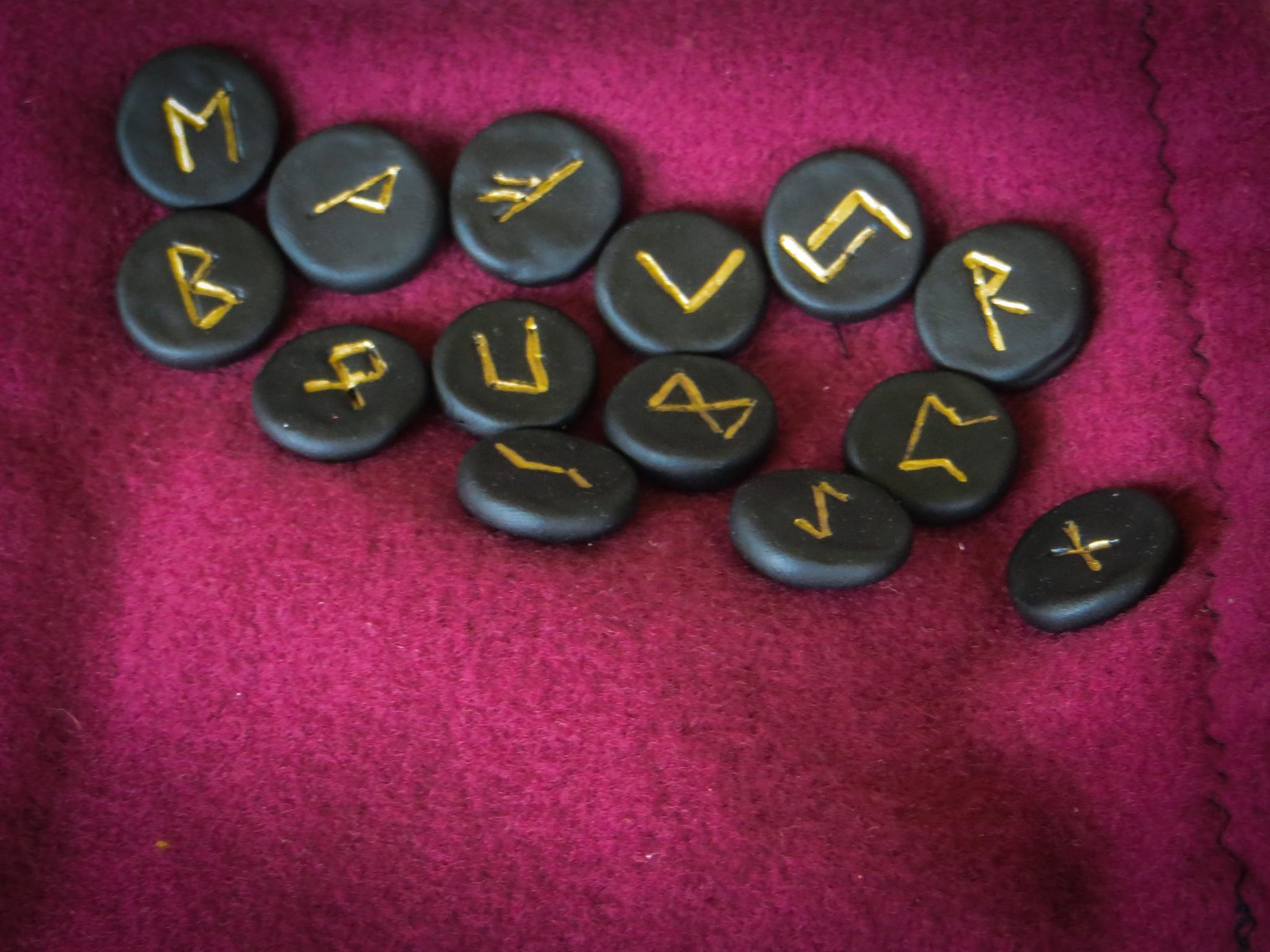The image depicted is a horizontal rectangular photograph showcasing a close-up of a magenta or fuchsia felt blanket that fills the entire frame. The blanket has a striking zigzag black stitch running from the top-right corner down to the bottom-right. Resting on this textured fabric are 14 black-painted, spherical stones, each adorned with a unique rune-like symbol engraved in a mustard yellow or golden color. These stones are roughly circular and arranged in a line starting from the mid-right, slanting upward toward the top-left corner. The red felt background features variations in its rosy red hue, adding depth to the image.